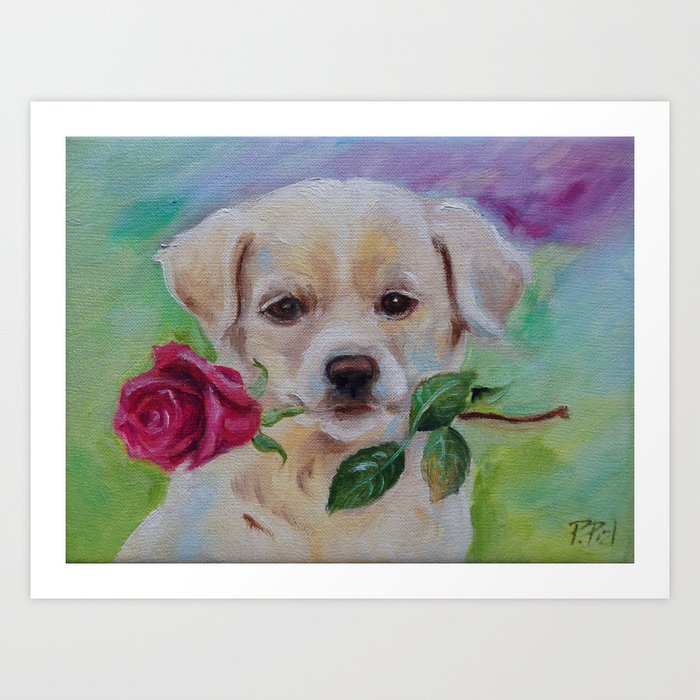The image is an oil painting of an adorable young puppy with light beige fur and white accents around its nose and mouth. The puppy, slightly older than a newborn but still youthful, gazes directly at the viewer with dark eyes and a simple, sad expression accentuated by its floppy, drooping ears. In its mouth, it holds a red rose, clasped midway along the stem, complete with several leaves. The background of the painting is a swirl of vibrant colors—green and blue along the sides, hints of yellow, and notably, purple concentrated in the upper right corner. The painting is on canvas, surrounded by a white border and prominently signed in the bottom right corner with the initials "PPD." The overall piece, which is displayed on a larger white wall, exudes a mix of whimsy and charm that would be fitting for an art gallery.